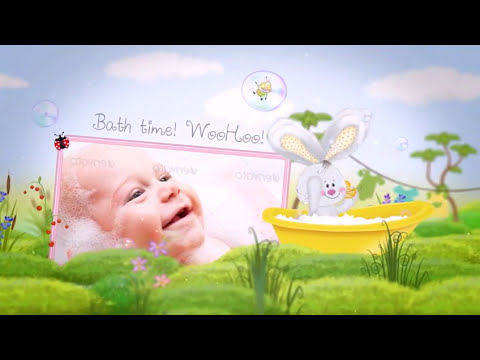The image depicts a cartoonish scene with a rectangular layout, bordered by thick black horizontal stripes at the top and bottom. In the center, a framed, colorful photo of a smiling baby is prominently displayed, angled slightly with soap bubbles around their bald head. The baby lies on its side against a white backdrop encased by a pink frame adorned with a ladybug in the top left corner. The setting features a vibrant sky with white clouds, and whimsical details such as green hills, scattered flowers, and blue blooms on the far left. To the right of the baby, a cheerful bunny with large ears, and a pink nose, sits inside a yellow bathtub filled with bubbles. The text “Bath time woohoo” appears in a playful font above the frame, enhancing the delightful and joyful ambiance of the scene.